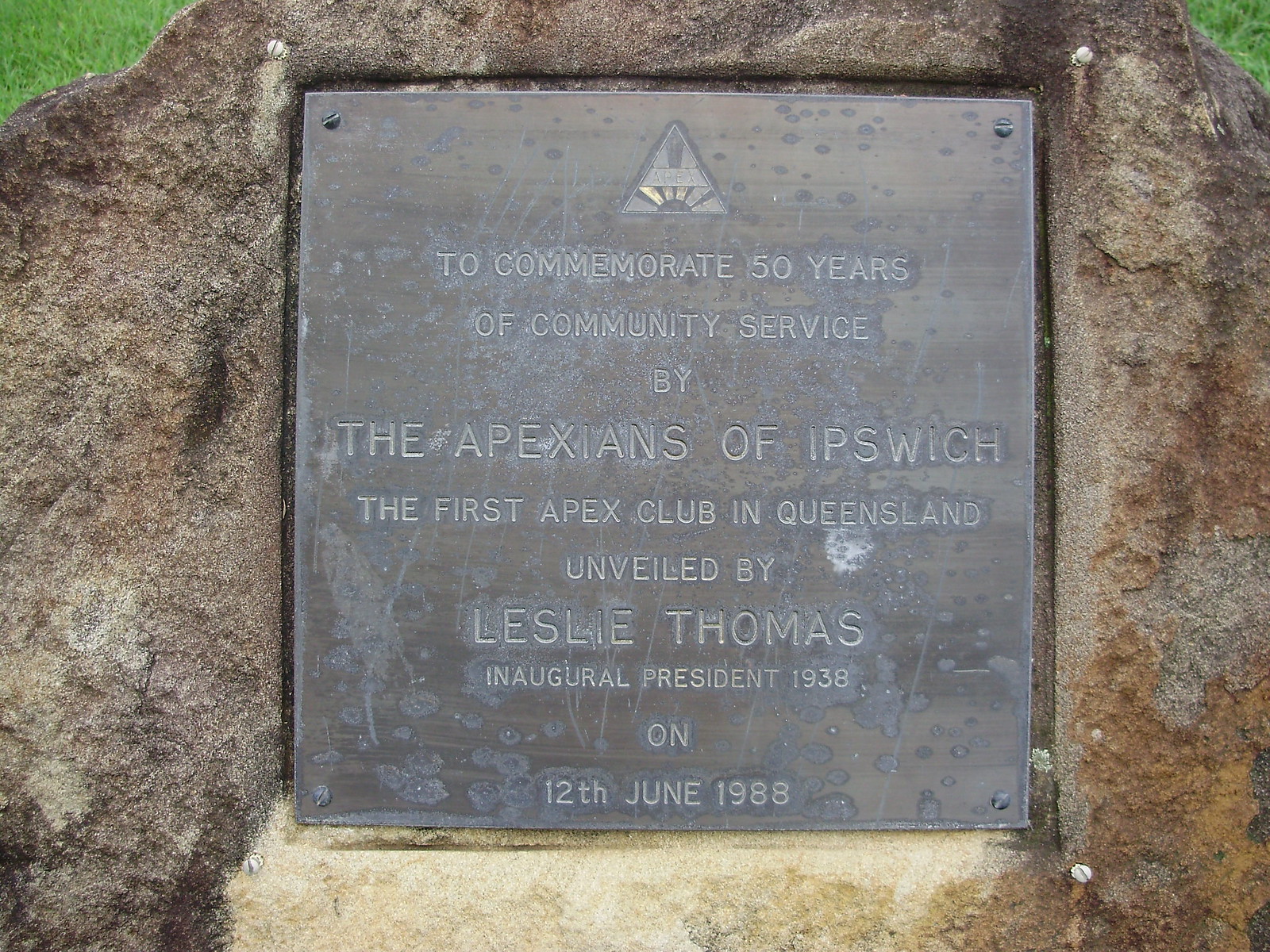The image features a commemorative plaque mounted on a piece of slate-colored stone. The plaque, affixed with metal screws, bears tan-colored engraved text that reads: "To commemorate 50 years of community service by the Apexians of Ipswich, the first Apex Club in Queensland, unveiled by Leslie Thomas, inaugural president, 1938, on 12th June 1988." The stone appears to be set outdoors against a backdrop of visible grass, suggesting it is an outdoor installation commemorating a significant milestone for the community.